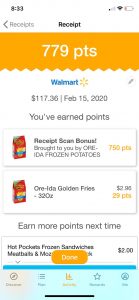A detailed close-up image of a Walmart receipt is shown. The receipt is timestamped at 8:33 AM on February 15, 2020. At the top of the receipt, the word "RECEIPT" is prominently displayed, followed by a points summary highlighted in white on an orange background, indicating "779 points." Beneath this summary, the iconic Walmart logo is clearly visible, accompanied by a total purchase price of $117.36.

The receipt details two items, albeit the name of the first item is blurred and cannot be distinctly identified. Despite the blur, it appears to be an order of frozen fries associated with O-R-E-I-D-A and worth 750 points. Next to it reads "Brought to you by O-R-E-I-D-A Frozen Potatoes." The second listed item is "O-R-E-I-D-A Golden Fries," with the cost partially blurred but discernible as $2.95. It specifies a quantity of 32 ounces and is worth 29 points.

At the top of the first item, there is a notation for a "Receipt Scan Bonus" worth 750 points. Near the bottom of the receipt are the words "Next Time" followed by promotional text mentioning "Hot Pockets Frozen Sandwiches Meatballs and Mozzarella." The bottom concludes with a button labeled "DONE" for exiting the scan receipt function.